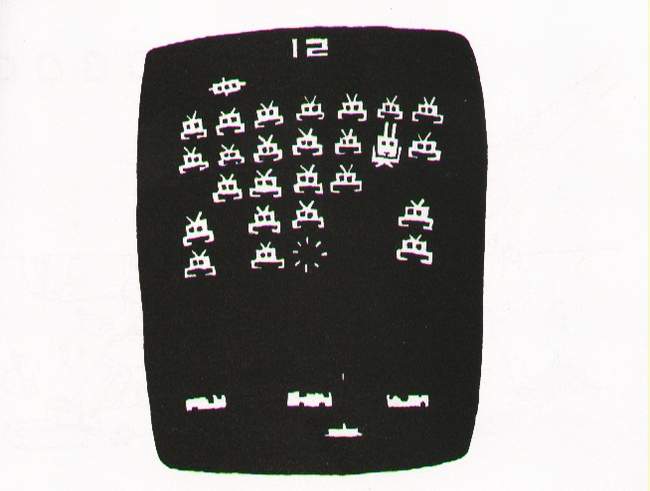The image depicts a classic screenshot from an early version of the Space Invaders video game, featuring a black background with a centered square object. At the top of this object, a white number 12 is prominently displayed. The scene is dominated by rows of white, alien-like creatures with antennas, reminiscent of early 1980s video game graphics. Positioned towards the bottom of the image are structures resembling little buildings or defensive blocks, several of which appear damaged or partially destroyed by the aliens' attacks. The aliens themselves are illustrated with simple shapes, primarily upside-down U's with two small eyes and a tiny V on top, characteristic of the game's minimalistic style. One alien is shown in the process of exploding, transforming into a sun-like shape. The overall design, though basic, effectively captures the intensity and iconic imagery of the classic arcade game.